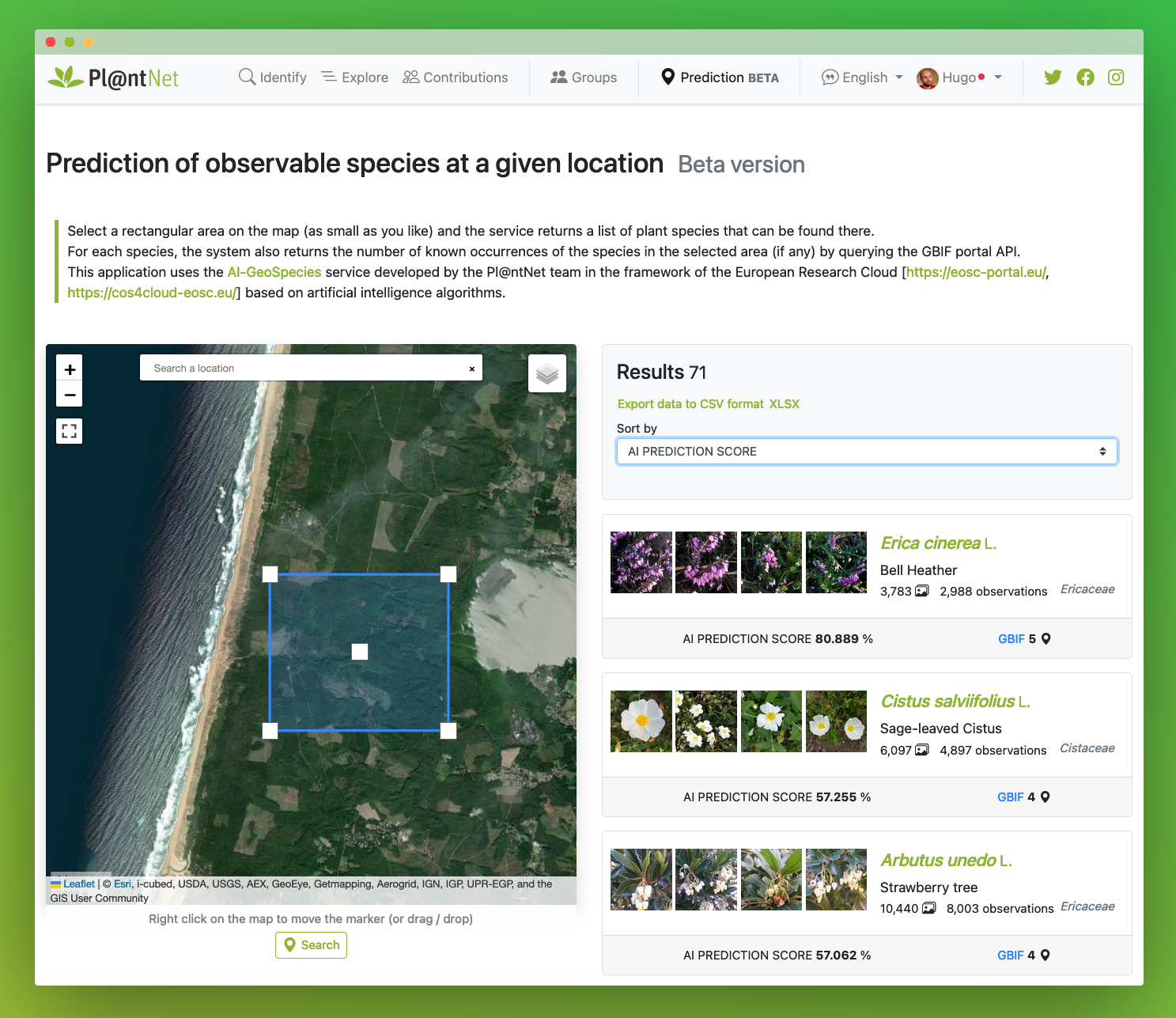This screenshot is from the PlantNet website, displaying a user interface designed to identify and explore plant species. At the top of the page, you see various navigational options such as "Identify," "Explore," "Contributions," "Groups," "Predictions," "Data," "English," and a user profile icon that reads "Hugo." Social media links for Twitter, Facebook, and Instagram are also visible.

The main feature showcased is the "Prediction" tool, which allows users to predict observable species in a selected geographical area. By drawing a rectangular selection on the map, the service generates a comprehensive list of plant species that are likely to be found in that location. Each listed species includes details about their occurrence and frequency in the chosen area. The platform provides high-resolution images, AI-generated prediction scores, and interactive map functionalities, enabling users to zoom in or out and move the markers with a right-click to refine their search.

This tool not only identifies plant species but also classifies and organizes them based on the input data, making it an indispensable resource for botanists, researchers, and nature enthusiasts looking to explore and document flora in specific regions.